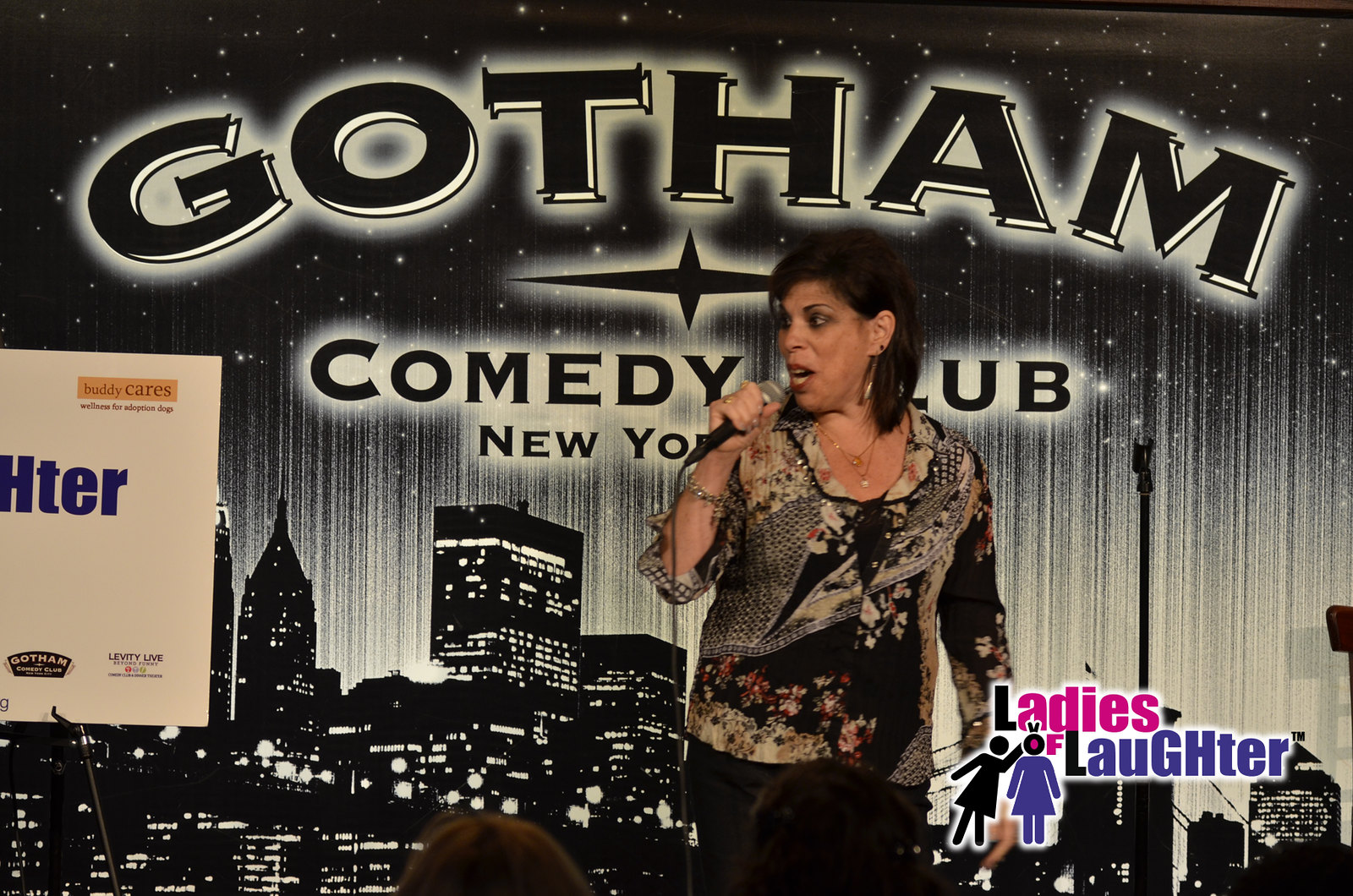In the image, a woman with dark hair, wearing a long-sleeved shirt and black pants, stands at the center holding a microphone. She appears to be performing, suggesting she is a comedian. The background features a faded, black-and-white depiction of New York City’s skyline at night, emphasizing the urban setting. Prominent text on the background reads "Gotham Comedy Club New York," indicating the venue. Additional text and a logo at the bottom right of the image identify the event as "Ladies of Laughter." The color contrast highlights the woman in vibrant color against the monochromatic backdrop. The setting is likely indoors at night, capturing the ambiance of a comedy club.